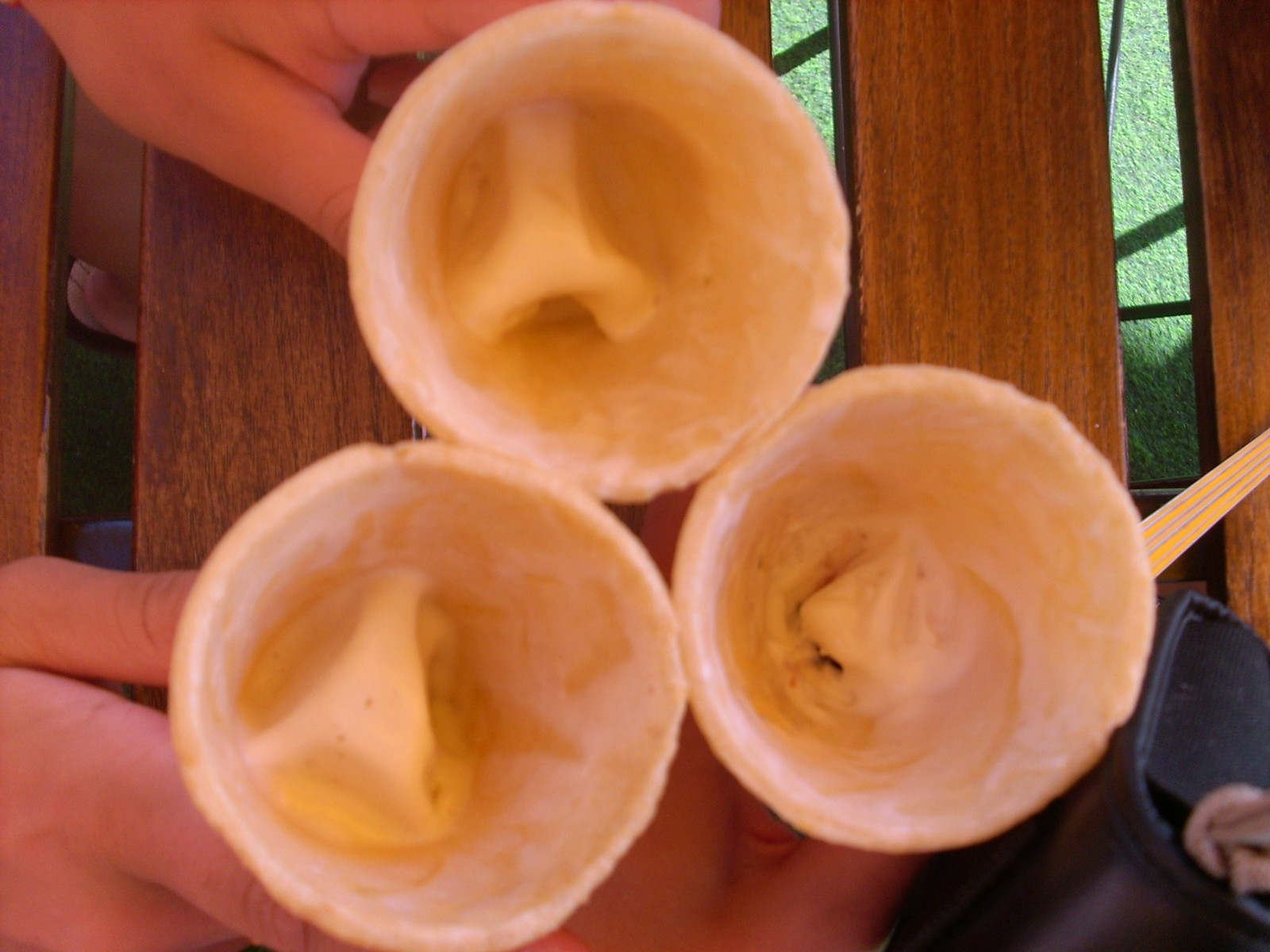This detailed photograph captures an overhead view of an outdoor setting, showcasing three partially-eaten ice cream cones held by two white hands. The ice cream cones, likely of the cake variety, are light beige, pink, and white, suggesting flavors like vanilla or a similar light ice cream. They are contained within slightly rough, styrofoam-like cups. The scene is set on a slatted picnic table through which astroturf, half bathed in sunlight and half in shade, is visible below. A person's leg can also be seen through the table slats, along with a small portion of a blue cloth napkin and a spoon, adding to the casual, summery atmosphere of the image.